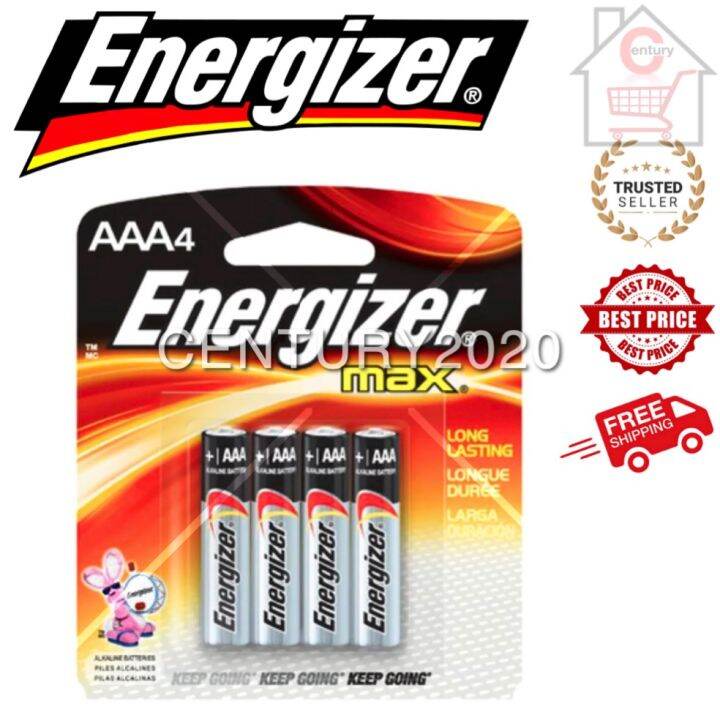A detailed caption for the described image:

---

A screenshot of an advertisement for Energizer Max AA batteries. The ad prominently features a picture of a house in the background. Overlaying the image, there is a brown circle with the text "Trusted Seller" and a red circle with the text "Best Price". Towards the bottom left, a red truck icon with white text reads "Free Shipping". The core product displayed is a pack of Energizer Max AA batteries, with "Energizer" written in white and "Max" in yellow. Descriptive text on the pack includes phrases such as "Long Lasting" and its French translation "Longue Durée". Additionally, the package showcases the iconic Energizer bunny playing a drum, accompanied by the slogan "Keep Going" in progressive shades of gray to black. The text "Century 2020" is also visible on the packaging. At the top of the image, there is a perforated hole indicating where the package would hang on a store's display hook.